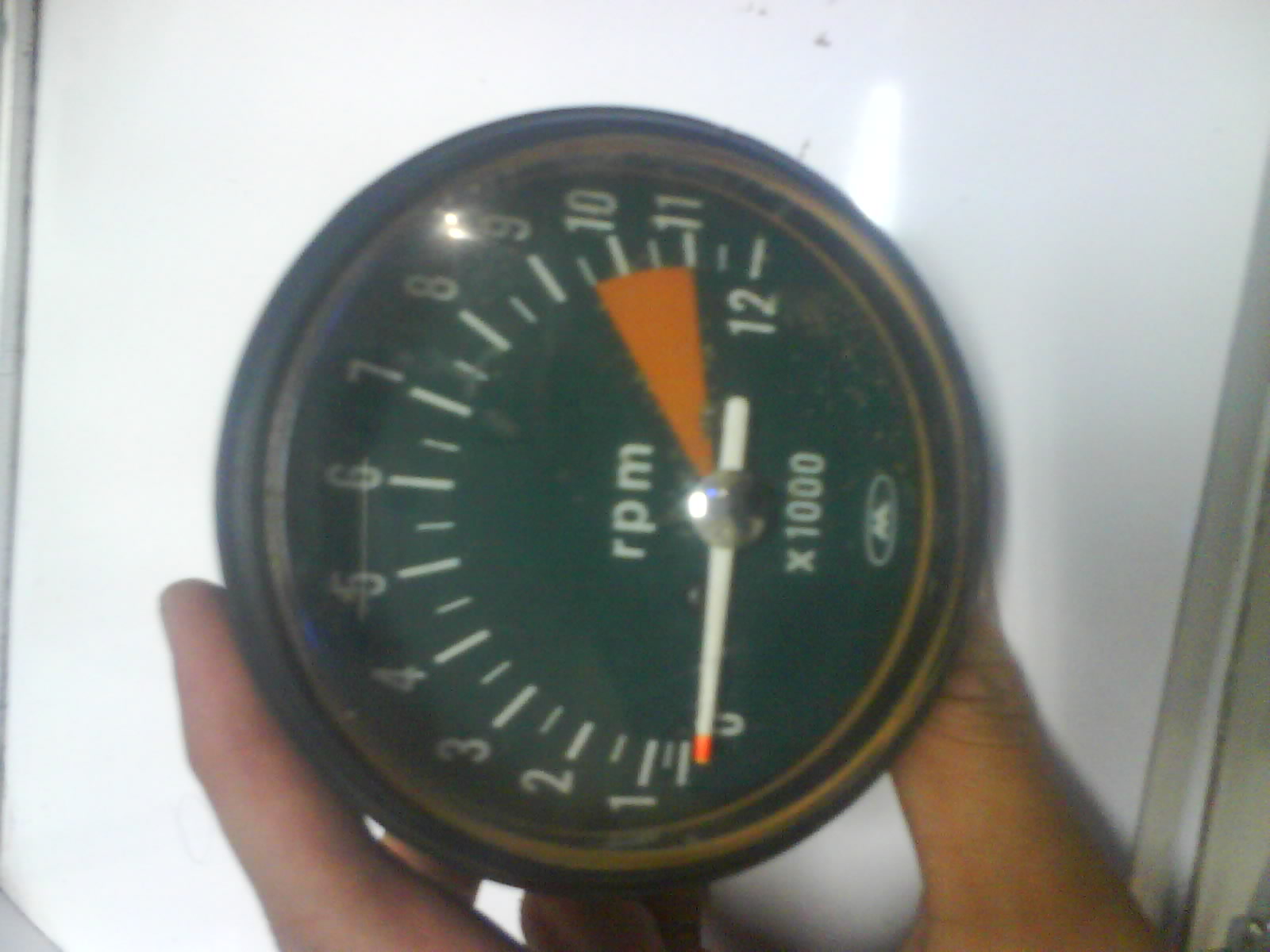The image is a close-up shot of a meter, specifically an RPM gauge, showcasing intricate details. The background of the gauge is a forest green color, providing a stark contrast to the white notches and numbers arranged in a circular pattern, ranging from 1 to 12. Prominently displayed in the center of the meter are the letters 'RPM'. Below this, a small, silver circle serves as the pivot point for the needle, which indicates the measured value. The needle is primarily white, with its tip colored in a striking neon orange for visibility. Underneath the central circle, the text 'X1000' is clearly marked, denoting the scale of measurement. Below this, there is a narrow, horizontal oval containing a faint symbol that is difficult to discern. The photograph appears to be taken by someone holding up the gauge, with part of their hand visible, stabilizing the device for the photo. The image captures the fine details and functional components of the RPM gauge effectively.